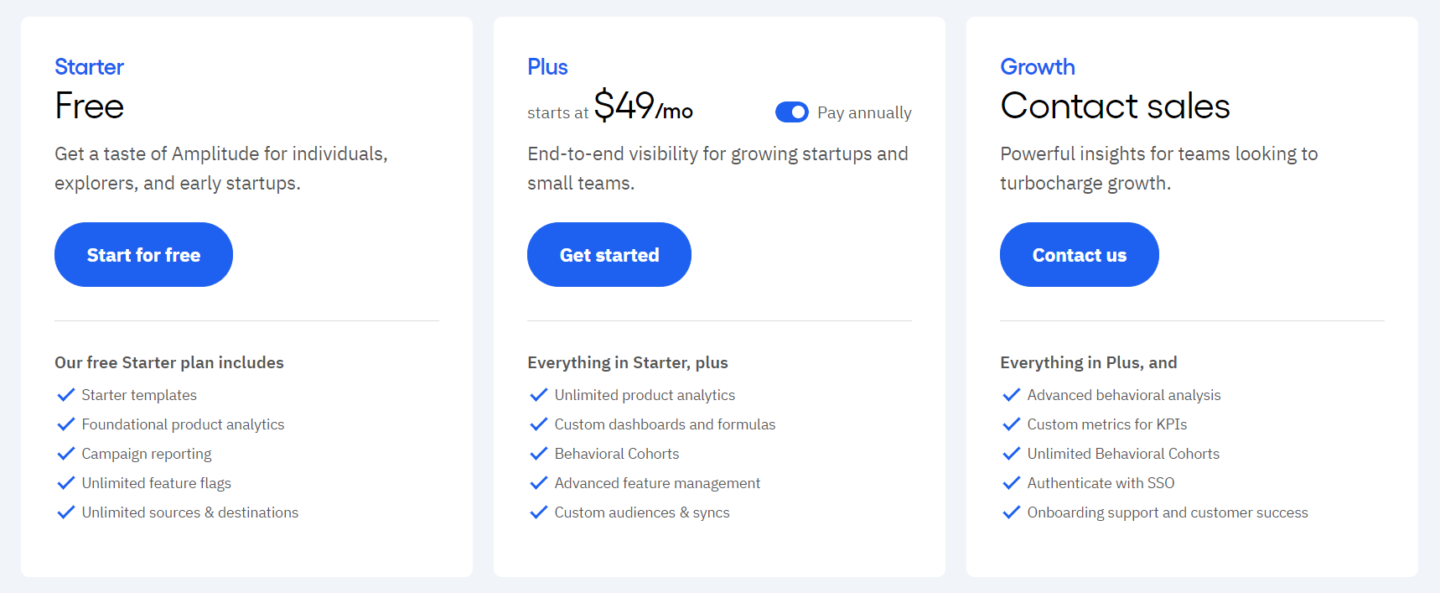This photographic image displays three square backgrounds aligned side by side, each presenting different subscription plan options.

The first background on the left showcases the "Starter" plan, with "Starter" written in blue text. Below, in black text, it reads "Get a taste of Amplitude for individuals, explorers, and early startups." A blue "Start for Free" button is prominently placed. The description beneath enumerates the features included: starter templates, foundation product analytics, campaign reporting, unlimited feature flags, and unlimited sources and destinations.

In the center, the "Plus" option is highlighted in blue, with a price of $49 per month billed annually. The accompanying description states, "End-to-end visibility for growth startups and small teams." A "Get Started" button is available for selection. The features listed include everything from the Starter plan plus unlimited product analytics, custom dashboards and formulas, behavioral cohorts, advanced feature management, and custom audiences and syncs.

The last section on the right is labeled "Growth" and offers a contact sales option. A "Contact" button is visible, inviting potential customers to reach out for further details.